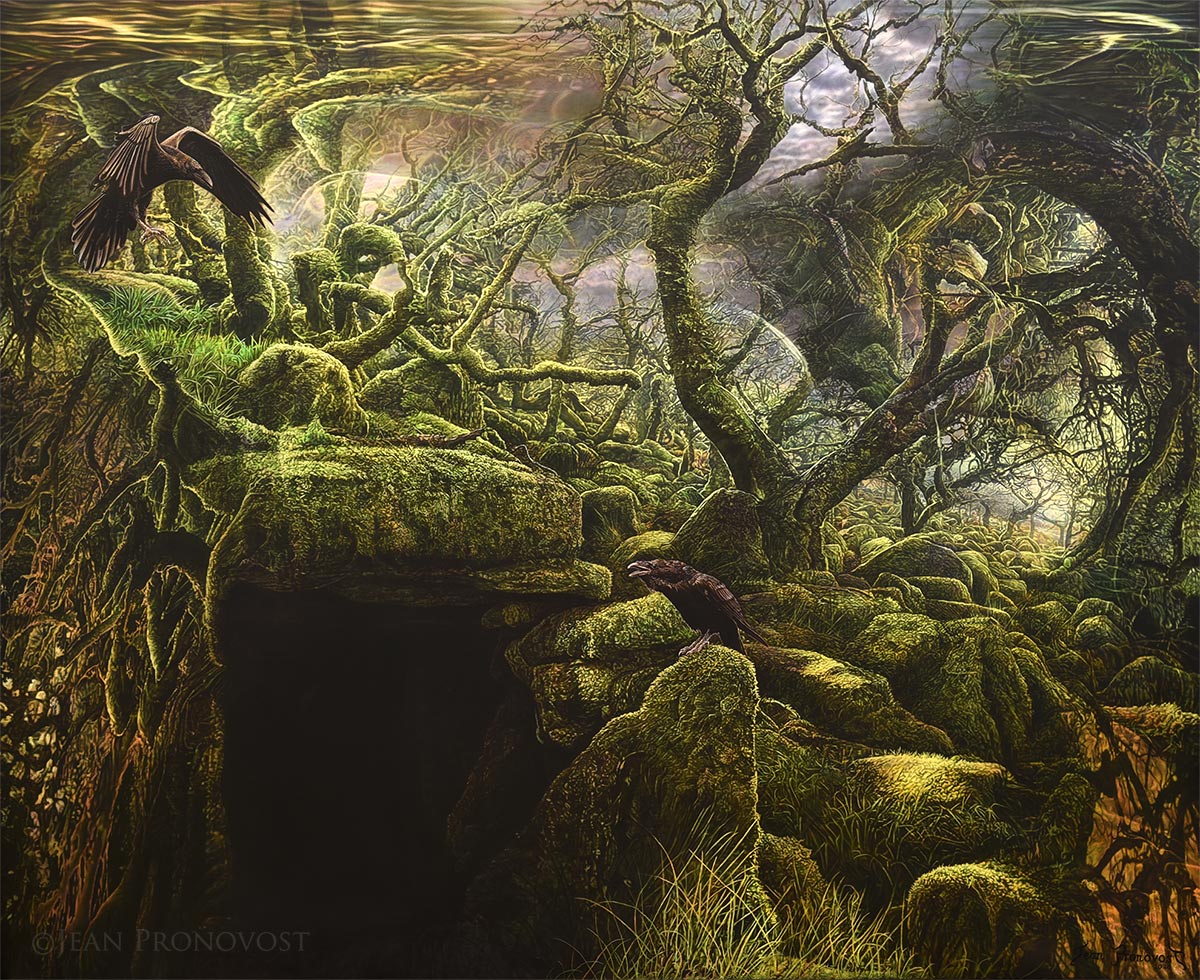The image is a detailed and moody illustration of a dark woodland or marsh scene, dominated by a large rocky outcropping that serves as the backdrop for a foreboding cave, its entrance shrouded in shadow. The rocks and numerous gnarled trees that rise in all directions are uniformly covered in a thick layer of moss, creating an eerie, overgrown atmosphere. Two large, black ravens add a menacing touch to the scene; one sits perched at the cave's entrance with its beak slightly open, while the other seems poised to take flight near the top left corner of the illustration. Green, noxious fumes emit from the cave, further enhancing the sinister feel. The top of the illustration shows a stormy or night sky, with hints of yellow fading to pink, possibly reflecting off a body of water, and cloud formations add to the dramatic tension of this fantasy setting. The intertwining branches of the trees and the shadowed details contribute to the complex, layered composition of the scene.